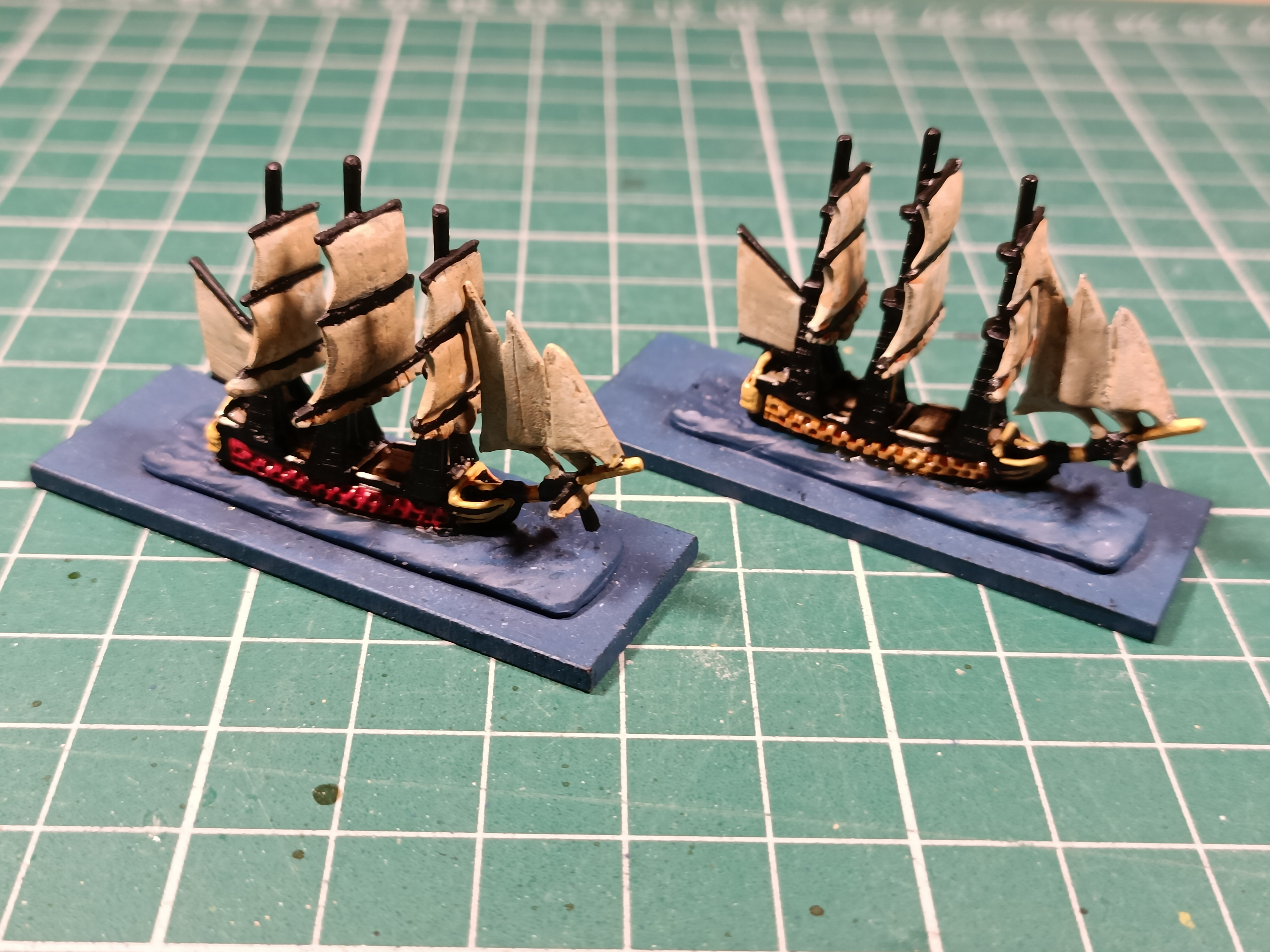The image features two impressive, miniature ship models placed on a turquoise green and white checkered, bathroom-like tile floor, which appears somewhat dirty. Each ship is displayed on a blue wooden plank platform. The ship on the left has a reddish-brown hue, while the one on the right is more yellow-brown in color. Both models resemble old pirate ships, with multiple tall masts reminiscent of those from the "Pirates of the Caribbean." These intricate models appear to be made of clay, with beige-colored sails adding to their detailed craftsmanship. The photograph powerfully captures the artistry and meticulous design of these miniature vessels, although the setting and purpose of the display remain unclear.